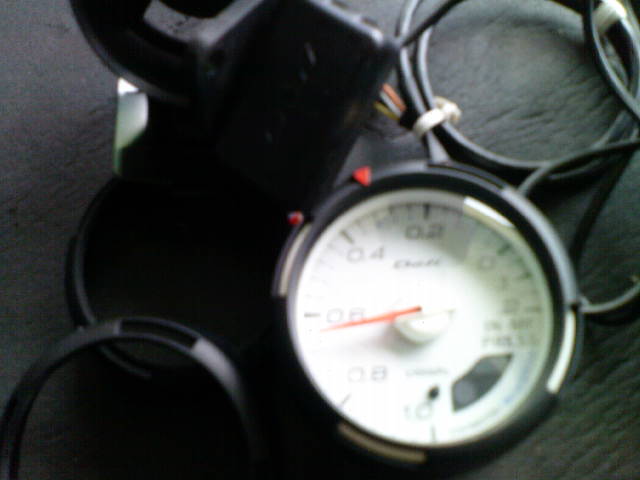The image features a gauge with a white face, marked with numbers ranging from 0.2 to 0.6. A red needle points to 0.6, indicating a reading. The gauge is encased in a black outer shell, which also features red markers. The image is slightly blurry, making it difficult to read the numbers clearly. 

In the bottom right corner of the gauge face, there is an unidentifiable black area, surrounded by some cables. Specifically, black cables looped together with a white band are visible in the top right portion of the image. To the left of these black cables, there are red, white, and yellow cables emerging from the black area, leading into a black plastic shell.

A light source from the top right corner illuminates part of the gauge and its surroundings, while the lower part of the image remains in shadow. A piece of plastic, part of the apparatus, can be seen in the bottom left. The entire setup rests on what appears to be a black, leather chair.